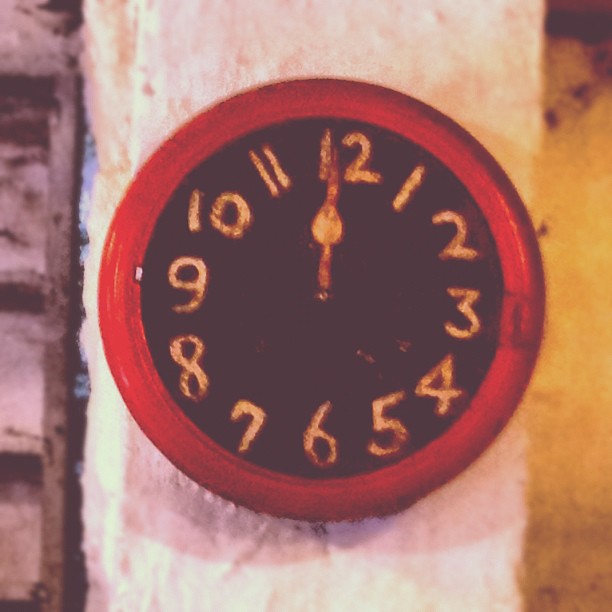This image showcases a clock mounted on a narrow, white wall with a somewhat blotchy texture. The clock is oriented vertically, occupying nearly the entire length of the wall. Its striking red frame encompasses a black clock face, which features bold yellow numbers arranged in a standard 1 to 12 configuration. The clock is distinctively minimalist, with only one short, yellow hour hand pointing directly at the 12, indicating it could be either noon or midnight. Absent is the minute hand, focusing attention entirely on the solitary yellow dial.

The surroundings add context but remain secondary to the clock. To the right, a yellow light casts a soft reflection on the wall, hinting at nearby illumination. On the left side of the image, an empty, gray shelf is partially visible but abruptly cut off by the photo's edge. The photo itself is slightly ambiguous in quality, leaving it open to interpretation whether it's a photograph or an artistic representation.